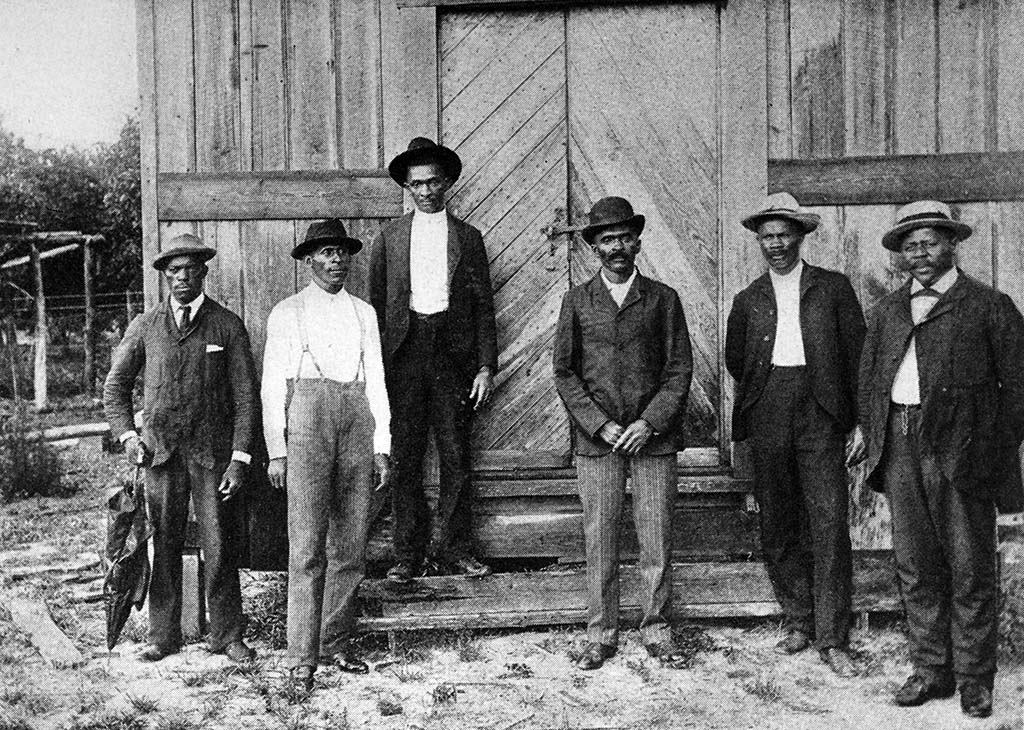In this black-and-white photograph from the late 1800s or early 1900s, six African-American men are posed in front of a wooden building that resembles a shack or shed. The structure, characterized by its absence of windows on this visible side, features wooden steps leading up to a double-sided door with a metal latch. The men are standing on a dirt or sandy ground punctuated by sparse patches of grass, with a few trees and wooden posts visible in the background. All six men are attired in old-fashioned suits and long pants, accessorized with hats; some are sporting suspenders, and their coats vary between buttoned and unbuttoned. The group exudes a serious demeanor, with some individuals looking directly at the camera while others glance to the side. One notable detail is a man holding an umbrella, which is pointed towards the ground.